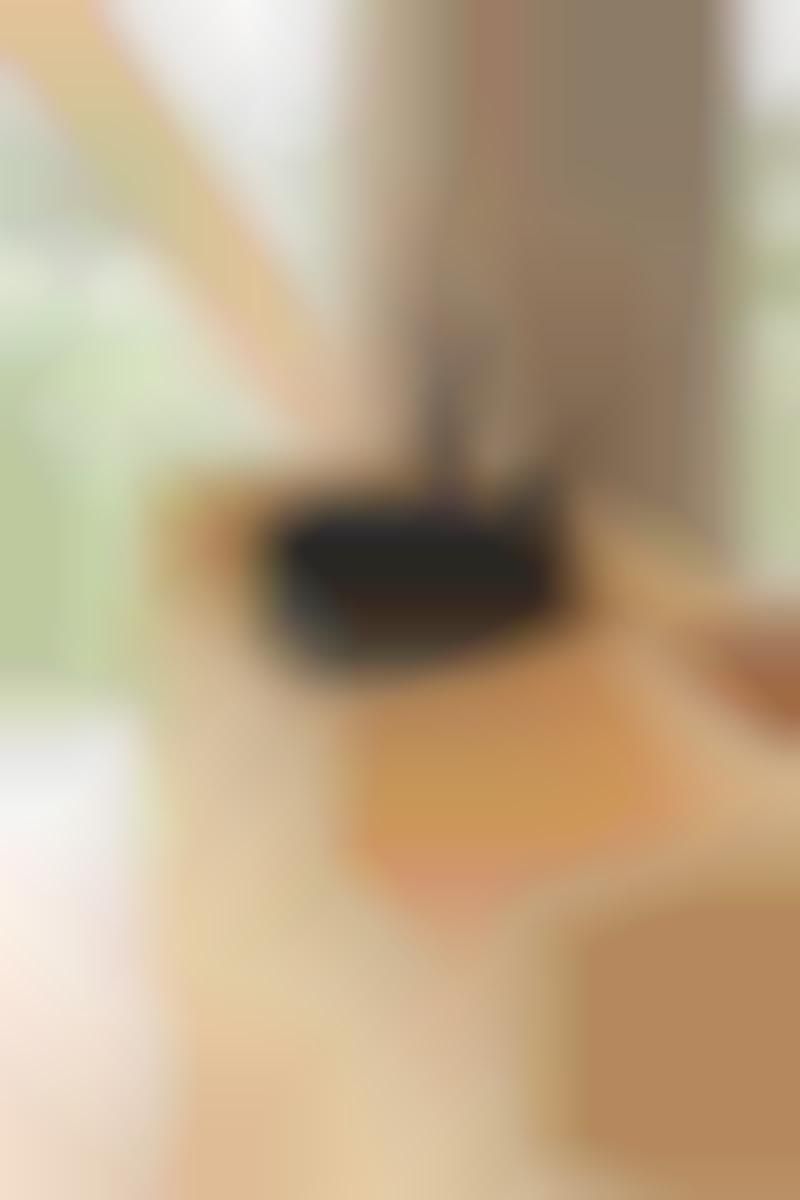The vertically oriented photograph captures an interior room featuring a light brown, unfinished wooden counter positioned in the middle to the lower right section. The counter, which appears to be a kitchen or work area, hosts a large, dark brown, circular sink basin with a glossy matte finish. A sleek, black faucet is mounted over the sink, though no water is running. The counter cupboards display medium brown knots, adding a rustic charm to the unfinished wood. In the background, two large, tall glass windows frame the upper left and upper right sides, revealing a lush, green yard with smaller green trees and grassy grounds. Brown drapes, neatly pulled back, adorn the corner between the windows. A visible beam runs diagonally across one of the windows, enhancing the architectural interest of the scene. The flooring in the room is a light, wood-like tile, complementing the overall light, earthy tones of the room.